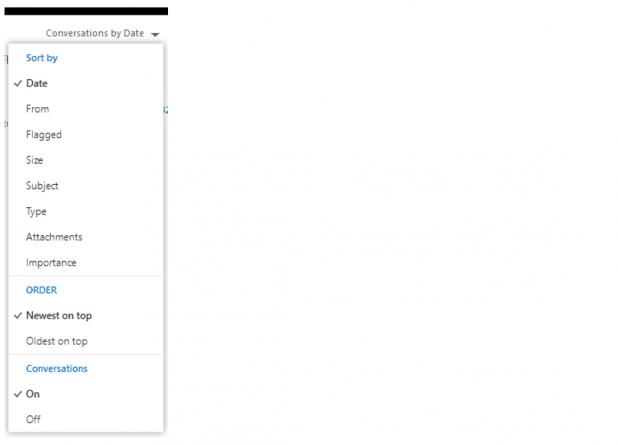The image depicts a filter settings page, likely within an email or messaging application. The background is entirely white, and the interface is clean and organized. 

At the top, there is a header titled "Conversations by Date" accompanied by a gray downward-facing arrow, indicating a dropdown menu. Directly below the header, there is a prominent blue "Sort By" button. 

The primary sorting option, "Date", is selected and marked with a black checkmark. Other available sorting options include "From", "Flagged", "Size", "Subject", "Type", "Attachments", and "Importance".

Below the sorting options, a blue "Order" button is visible. Users can choose to display conversations with "Newest on Top" or "Oldest on Top". Adjacent to this, there is another option titled "Conversation" with toggles for "On" or "Off", currently marked with an "On" checkmark.

The text on this page is predominantly black, with some elements highlighted in blue. At the very top of the image, a thin black bar stretches across the width, suggesting this is part of a larger application interface with multiple settings and options available. This is a single page of filters within the broader app or website.